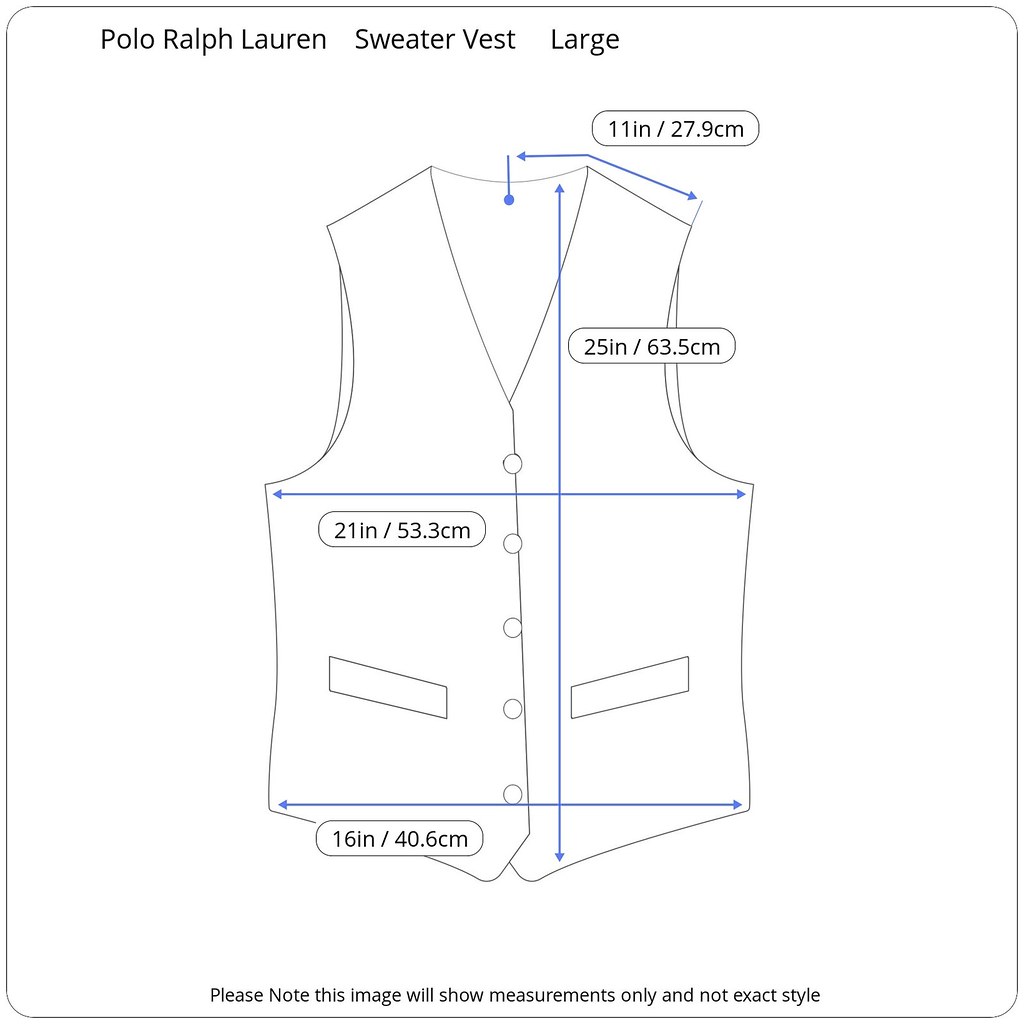This is a detailed digital square image of a pattern for a sewing project, specifically for a Polo Ralph Lauren sweater vest in a large size. The image is bordered by a thin black line with rounded corners. At the top, there is plain dark gray text that reads "Polo Ralph Lauren Sweater Vest Large." 

In the center, there is a simple black and white line drawing of a sleeveless vest with a V-neck, five buttons down the middle, and pockets on both sides. The drawing is annotated with several blue arrows indicating measurements. Two horizontal arrows provide the width at various points, including from under the left arm to under the right arm (21 inches or 53.3 centimeters) and from the bottom hem on the left to the right (16 inches or 40.6 centimeters). A vertical arrow indicates the height from the top to the bottom of the vest (25 inches or 63.5 centimeters). Another arrow goes from the right shoulder to the middle, indicating a measurement of 11 inches or 27.9 centimeters. 

At the bottom of the image, there is a small black text note stating, "Please note, this image will show measurements only and not exact style."